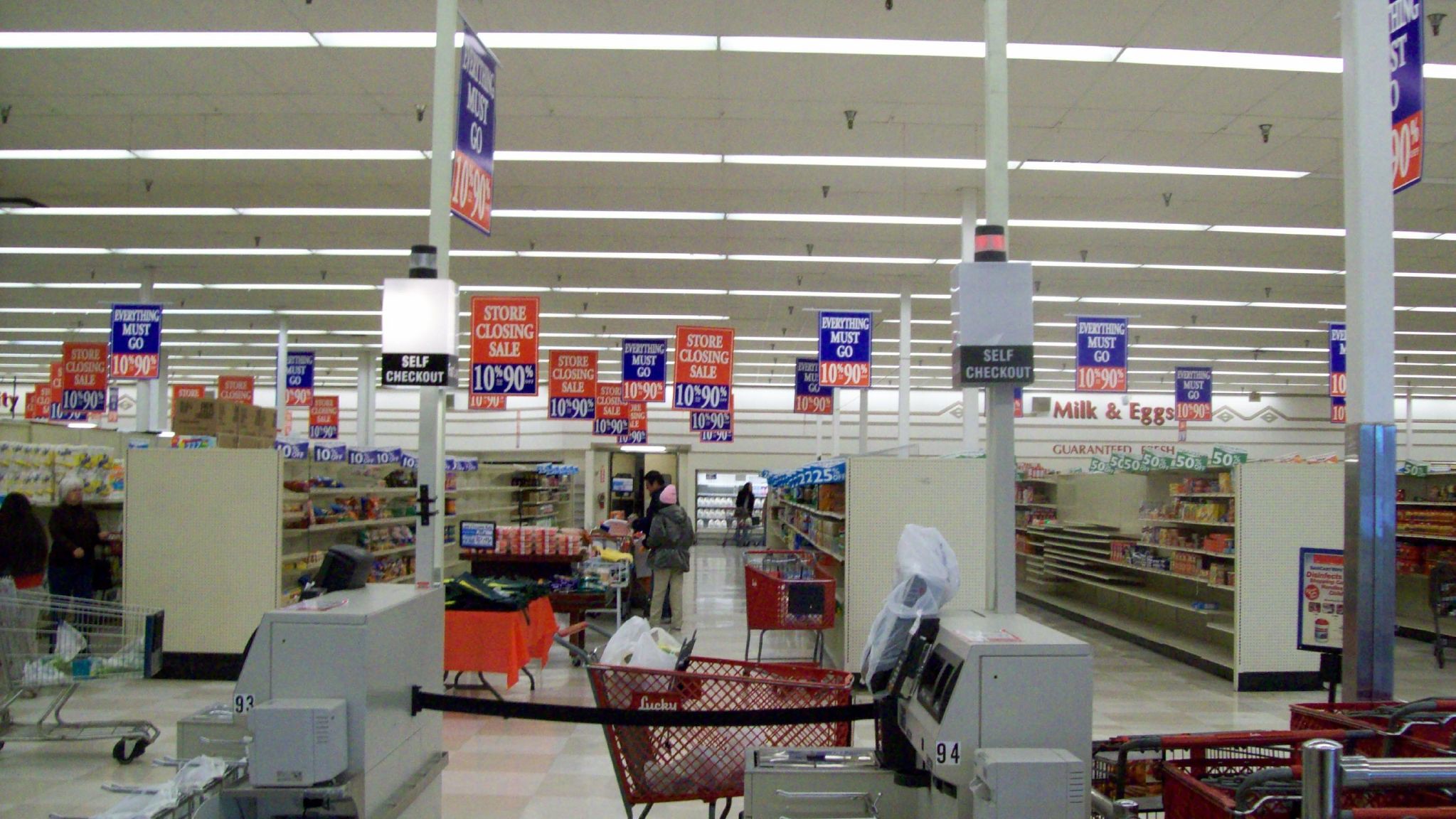This image captures a department store on the brink of closing, characterized by its desolate aisles and sparse shelving. Rows of vertical aisles crisscross the store, with mostly barren shelves that hold a few remaining food products. Shoppers navigate the store with red and silver shopping carts, adding to the melancholic scene. The self-checkout area, distinguished by white registers, is visible in the foreground. Hanging from the ceiling, a multitude of blue and red signs proclaim, "Before Closing Sale: 10 to 90% Off, Everything Must Go." The ceiling is also adorned with a grid of horizontally aligned lights, illuminating the scene with an almost stark brightness.